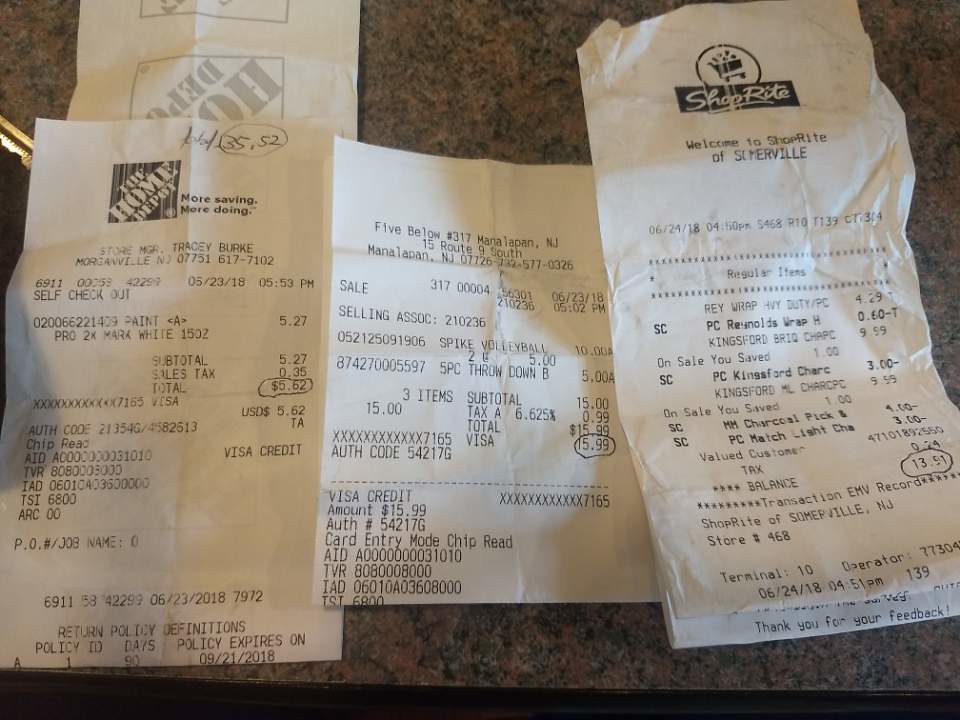This detailed color photograph features three store receipts placed on a zoomed-in dark brown, mottled marble surface, which displays intricate patterns of black and lighter golden brown hues. At the bottom of the image, a black shadow is visible, adding depth to the composition. 

Starting from the left, the first receipt is folded with the visible back end displaying lighter grey letters written diagonally, forming a square design. This receipt is from Home Depot, showcasing a black box with "The Home Depot" in white text, and underneath, the slogan "More saving. More doing." in black letters. Notably, written at the top in black pen is the total amount of $35.52, circled, along with the purchase date 05/23/18 at 5:53 p.m., and a self-checkout annotation. A small shadow crosses over the left edge of this receipt, and a tiny bit of gold is visible in the upper left corner. 

The middle receipt, smaller in size, is from Five Below, transaction number 317 in New Jersey, featuring a price of $15.99 circled. There is also an indication of a Visa credit card entry. 

The right-most receipt is from ShopRite of Somerville, with a circled price of $13.51. Above this is a black and white shopping cart logo. 

Significantly, a tiny part of a key is visible, peeking out just below the left receipt from Home Depot, hinting at an everyday context of these transactions.